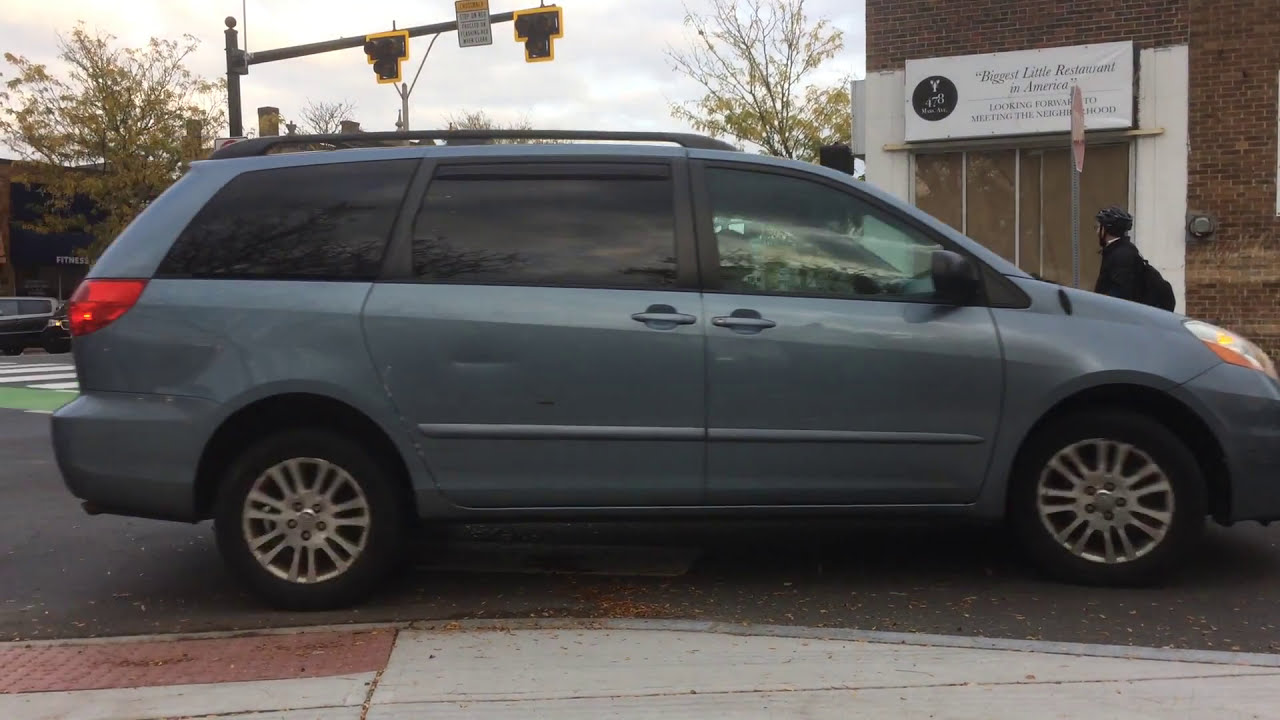The image shows a side profile of a gunmetal-gray minivan parked along a street next to a sidewalk made of mostly concrete with some red patterned stones. The taillights and headlights of the minivan are illuminated, and there are noticeable dents on both the front and back doors. In the upper part of the image, a streetlight pole extends horizontally and includes traffic lights and a yellow and white sign that appears to be a school sign. Across the street, there is a brown brick building with a white banner that reads, "Biggest Little Restaurant in America" in black print. A man wearing a bike helmet, dark clothing, and a black backpack is seen walking towards the left side of the image behind the minivan. The sky is light blue with scattered clouds, and sparse-leaved trees are visible in the background.